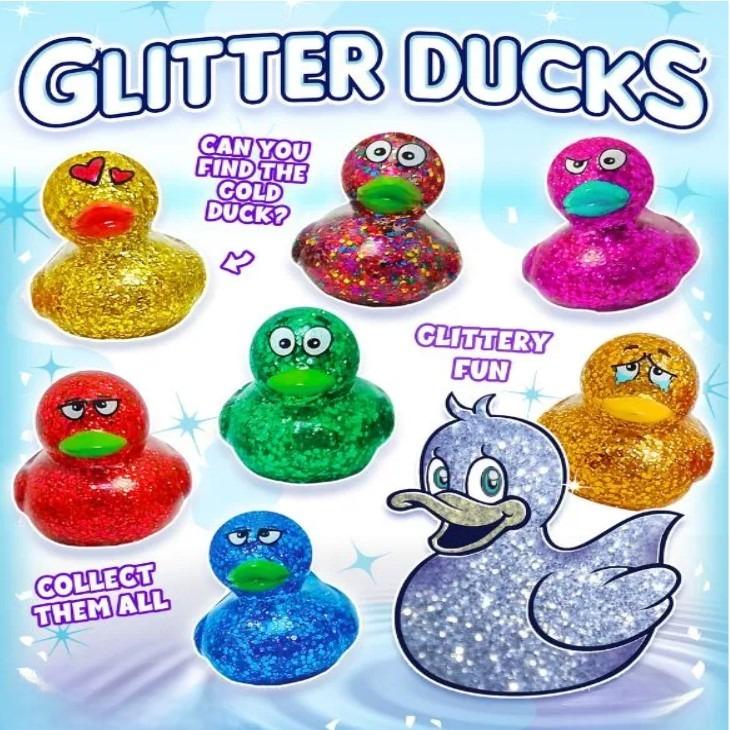This color image serves as an informational slide or advertisement for "Glitter Ducks," a collection of vibrant, glittery toy ducks. The top of the slide prominently features the title "Glitter Ducks" in white text with a blue outline. Among the ducks, arranged in approximately two rows, are various colors, including a gold duck accompanied by the text "Can you find the gold duck?" in white with a purple outline. The glittery ducks come in a multitude of colors: a multicolored duck adorned in red, pink, yellow, and orange hues; an angrily expressive bright pink duck; a standard yellow duck; a surprised-looking green duck; a fed-up red duck; an unhappy blue duck; and an extremely happy silver duck with a smile. Additionally, there's a cartoon version of a duck in the lower right corner, featuring a white body with red, blue, and white dot patterns. The background is a light blue water scene sprinkled with small blue stars. Other text phrases scattered throughout the slide include "Glittery Fun" and "Collect Them All."